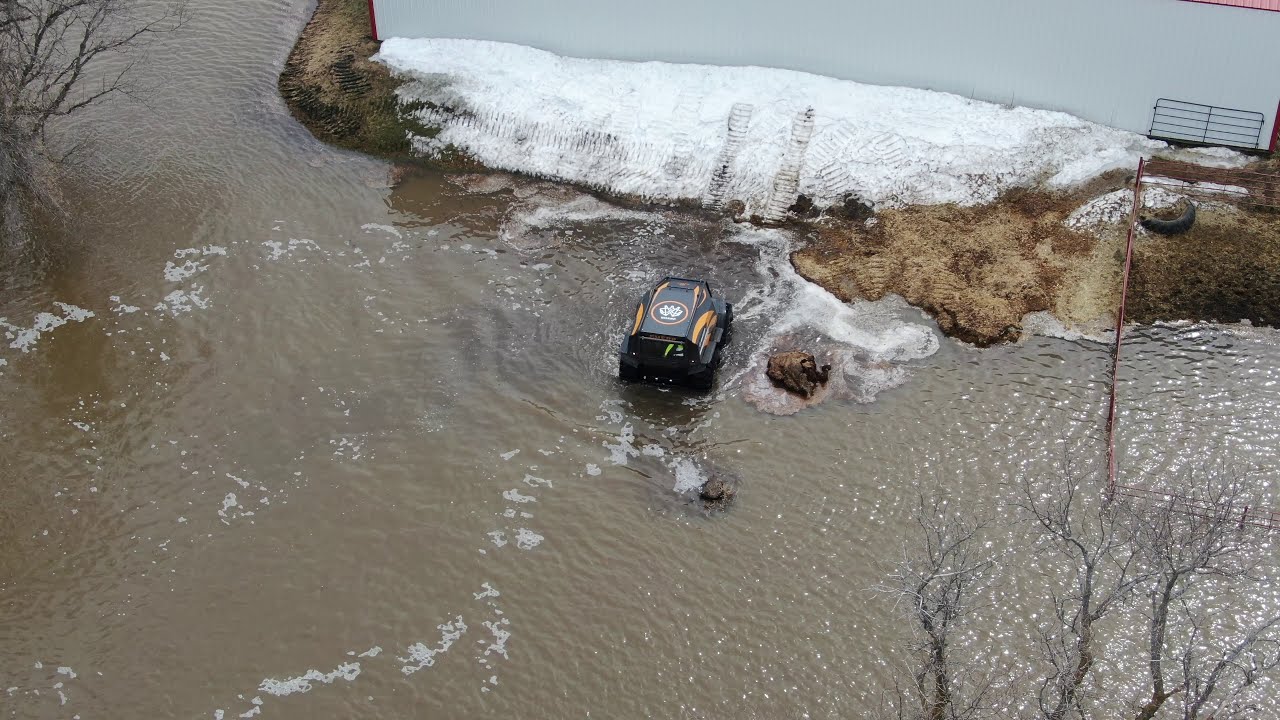This aerial photograph vividly captures a winter scene dominated by a serene body of water, likely a small lake or flooded area, covering roughly 85% of the frame. The remaining landscape includes scattered patches of snow and bare terrain. A black all-terrain vehicle with yellow and potentially green or orange accents is prominently featured, either partially submerged or just beside the water's edge, its large tires either obscured or suggesting partial immersion, supporting the idea that it is dealing with a flood situation.

Visible tracks in the snow indicate the trajectory of the vehicle, possibly suggesting it has been repeatedly moving back and forth over the same path. The faint outlines of additional elements include craggly, leafless branches sprawled across the scene, typical of vegetation found near waterways, and a weathered fence segment in the upper right corner. The barren top of a tree peeks into the lower right of the image, further emphasizing the wintry, stark nature of the environment.

The main color palette of the image consists of tans, browns, whites, and blacks with hints of yellow, perfectly encapsulating the blend of natural and artificial elements in this chilly landscape. There are no signs of human presence, fish, or boats, reinforcing the solitary and somewhat desolate atmosphere conveyed by the photo.